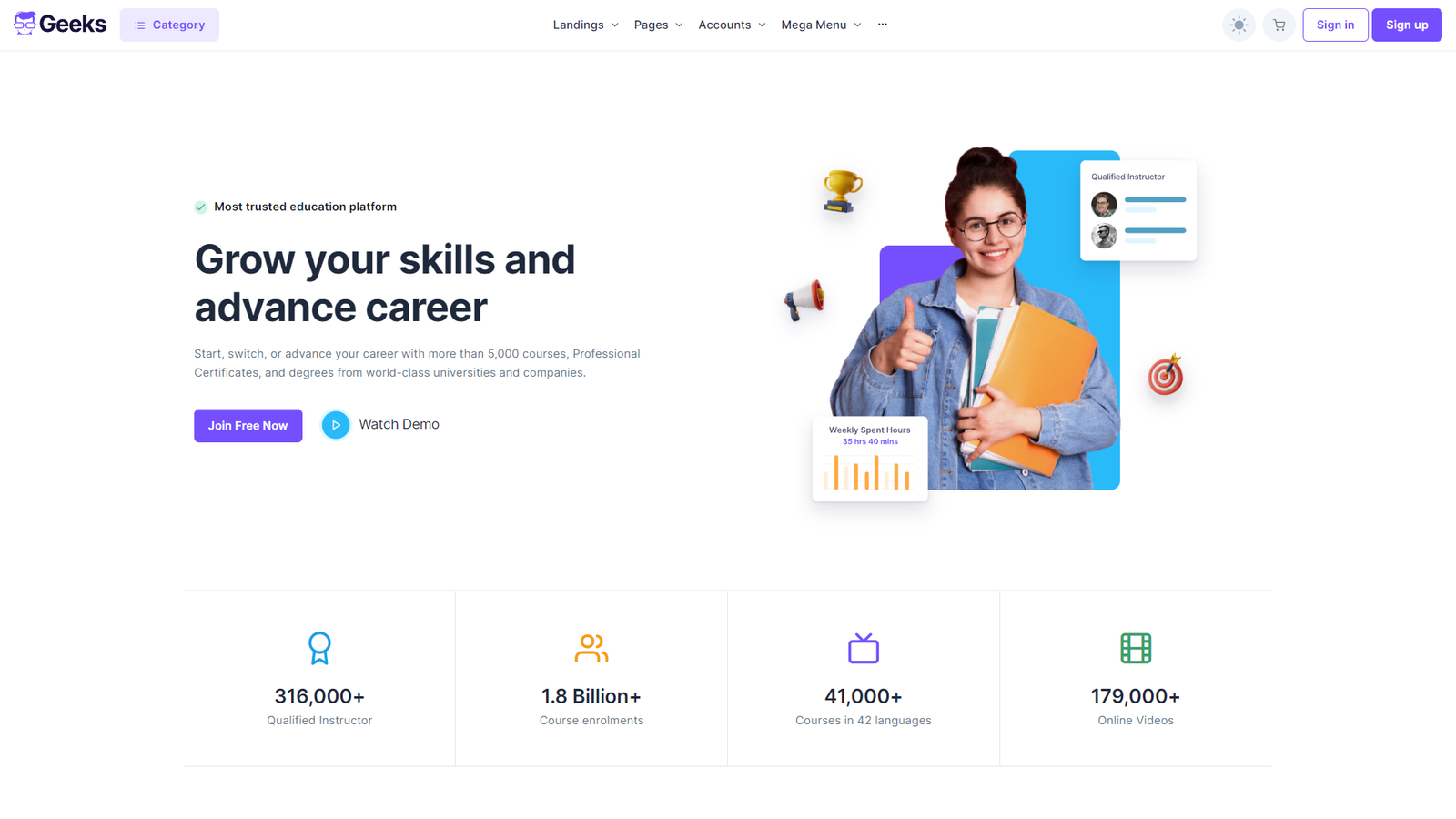A detailed screenshot of a website is displayed with a clean white background and a horizontal landscape layout. In the top left corner, the word "Geeks" is prominently featured. Next to it, there is an image of a person with purple hair and glasses. Below this image, within a gray box, a category label is present.

The central portion of the top header features several menu options, including "Landings," "Pages," "Accounts," and "Mega Menu." On the top right corner, there are "Sign In" and "Sign Up" options, with "Sign Up" highlighted in purple.

In the main section of the page, large black text reads "Grow your skills and advance your career." Below it, there is a subheading stating, "Start, switch, or advance your career with more than 5,000 courses, professional certificates, and degrees from world-class universities and companies." The call-to-action buttons are prominently displayed: "Join Free Now" in purple text and "Watch Demo" inside a blue circle. An endorsement above these buttons reads, "Most trusted education platform."

Below the text, an image depicts a woman with glasses and her hair tied up in a bun, wearing a denim jacket. She is holding several folders in her left hand and giving a thumbs up with her right hand. Surrounding her are icons of a trophy, megaphone, and bullseye.